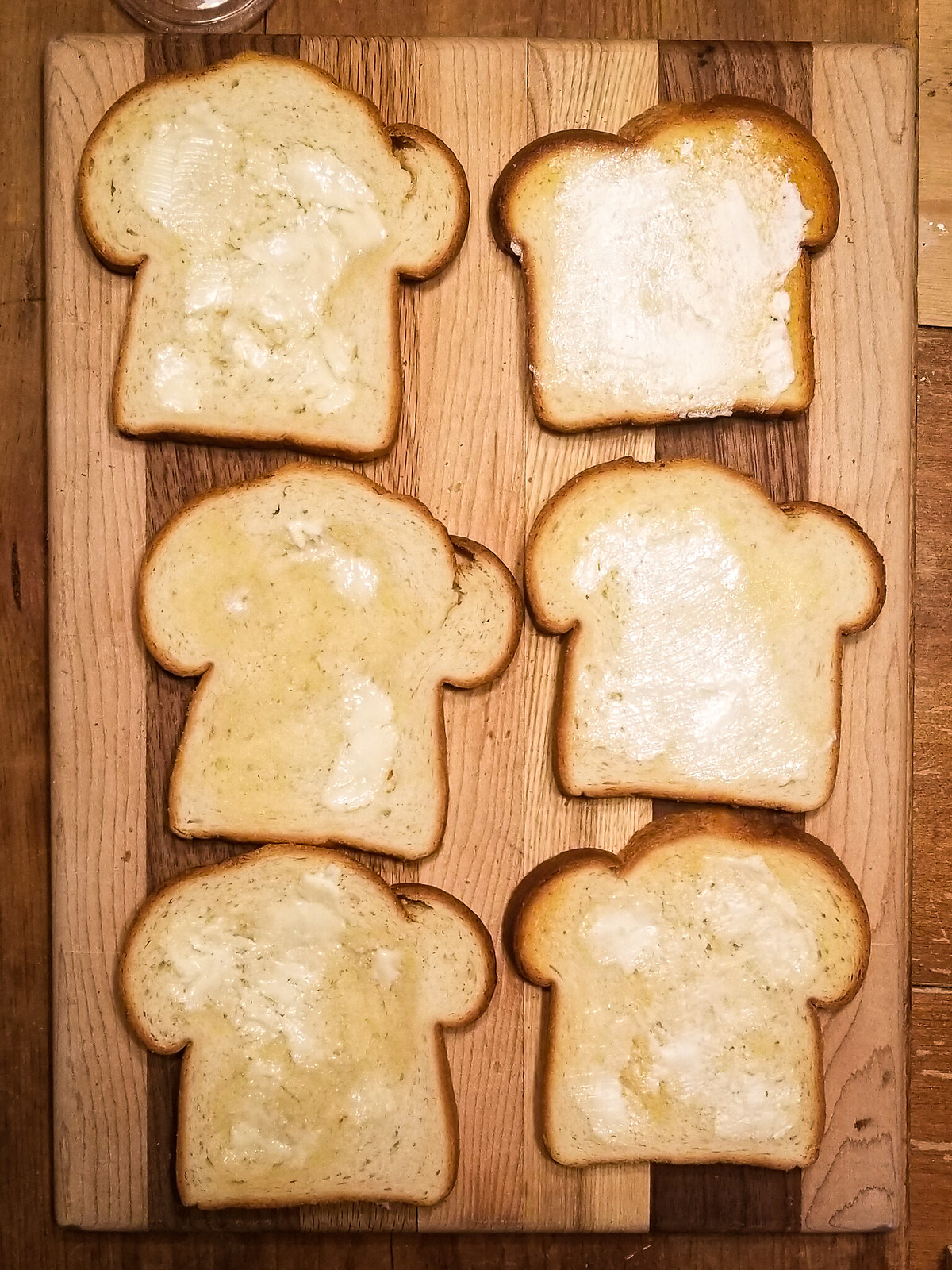This is a detailed colour photograph taken from a top-down, close-up perspective. The image showcases six slices of toasted bread arranged on a wooden cutting board with vertical slats. The cutting board, mainly comprised of light wood, features two distinct darker wooden slats—the second from the left and second from the right. The bread slices are organized into three rows of two, occupying a position on a surface with assorted coloured wooden panels and encircled by a wooden brown edge.

Each slice of bread, slightly golden from toasting, varies in its coverage of a white buttery spread, which is partially melted and visible where it has soaked into the toast. Notably, the upper right slice has the most spread, with the slice directly beneath it having the second most. The slices at the bottom and on the right side have noticeably less spread. Despite the subtle differences, all slices appear uniformly shaped like a chef's hat, suggesting they were cut from the same loaf of bread that likely required self-slicing.